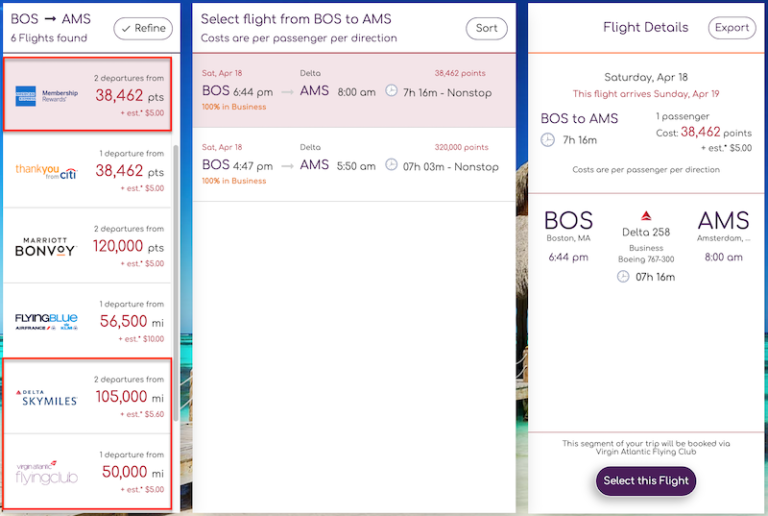The image displayed on the computer screen features a blue outdoor-themed background, although it is barely visible. Dominating the screen are three vertically-oriented, rectangular boxes with a white backdrop; the middle box is noticeably thicker than the two adjacent ones, which are almost identical in size. 

The content within these boxes lists travel itineraries starting from the airport code BOS (Boston) to AMS (Amsterdam). A heading indicates that six flights have been found, and a "Refine" button is available next to this summary.

Under the summary, the first itinerary is an offer from American Express, showing 38,462 points. The second listing is from Citibank's ThankYou program, also for 38,462 points. Following this is an offer from Bonvoy requiring 120,000 points. FUMG Blue is listed next with 56,500 points. Delta SkyMiles requires 105,000 miles, and finally, Flying Duo offers a rate of 50,000 miles.

In the middle section, there is a prompt to select a flight from BOS to AMS, with costs specified per passenger per direction. An "Sort" button is available for sorting the options presented. Beneath this, two different itineraries are offered for selection.

On the far right, the vertical box contains detailed flight information, an "Export" button, and additional itinerary specifics. Finally, at the very bottom of this box, there is a prominently displayed purple button with the text "Select This Flight" written in white.